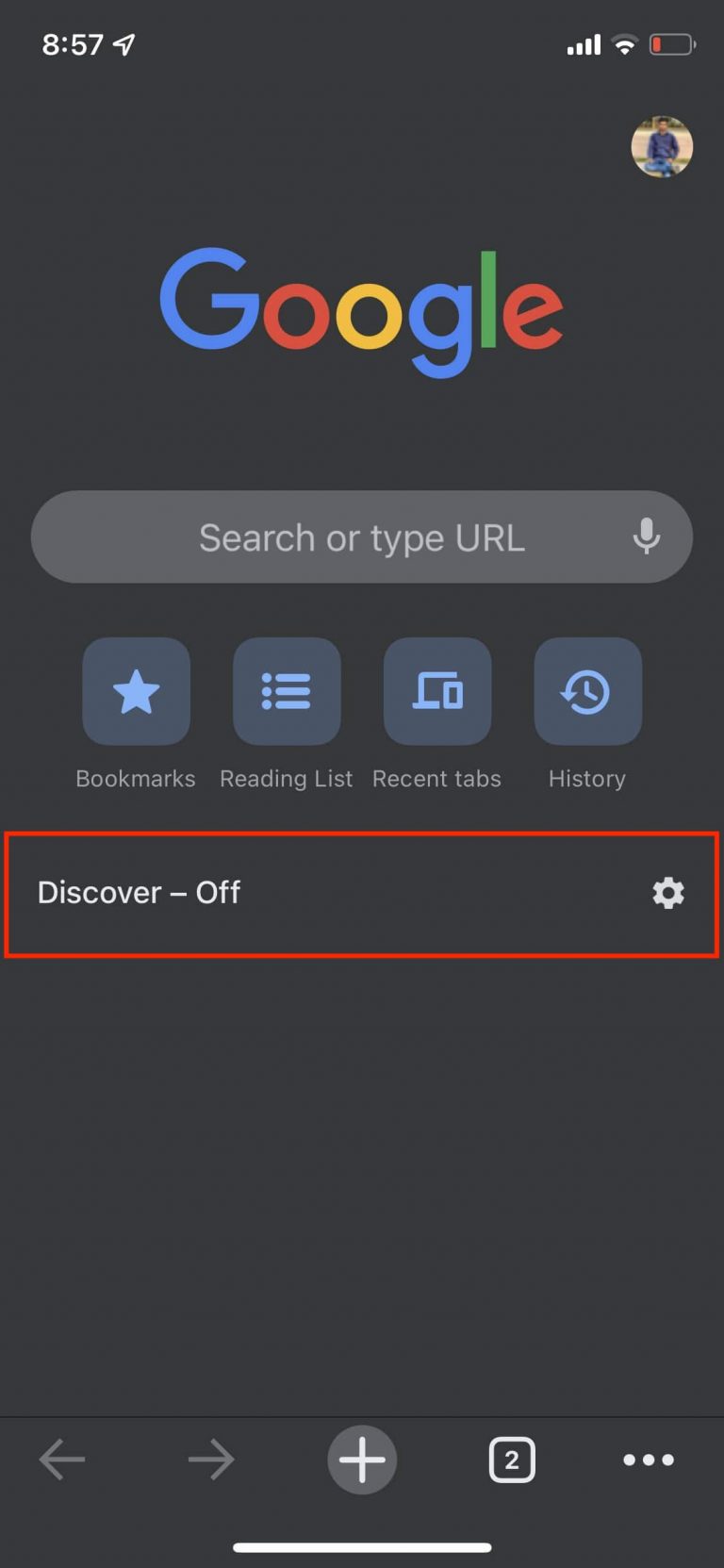The image displays a smartphone screen with various indicators and app elements visible. At the top, the screen shows the time as 8:57 and features four bars of signal strength, a Wi-Fi status icon, and a nearly depleted battery indicator. Below these indicators, there's a circular icon containing a picture of a person dressed in a blue shirt and blue jeans. The person's dark hair makes it difficult to determine their gender.

Directly beneath this image, the word "Google" is displayed in large, colorful letters (blue, red, yellow, and green). Below this, the search bar reads "Search or type URL" and features a grey microphone icon on the right side. Beneath the search bar, several menu options in blue are listed: "Bookmarks" with a star icon, "Reading List" with three horizontal lines and dots, "Recent Tabs" with a computer icon, and "History" with a backward-facing arrow. Additionally, there is a “Discover off” notice in a red square with a settings icon to its right, which is colored black.

Towards the bottom of the screen, a black navigation bar contains a back arrow, a forward arrow, a plus sign, a square with the number 2 inside it, and three vertical dots serving as a menu icon. Below this navigation bar, a thin white line is visible, completing the elements shown on the screen.